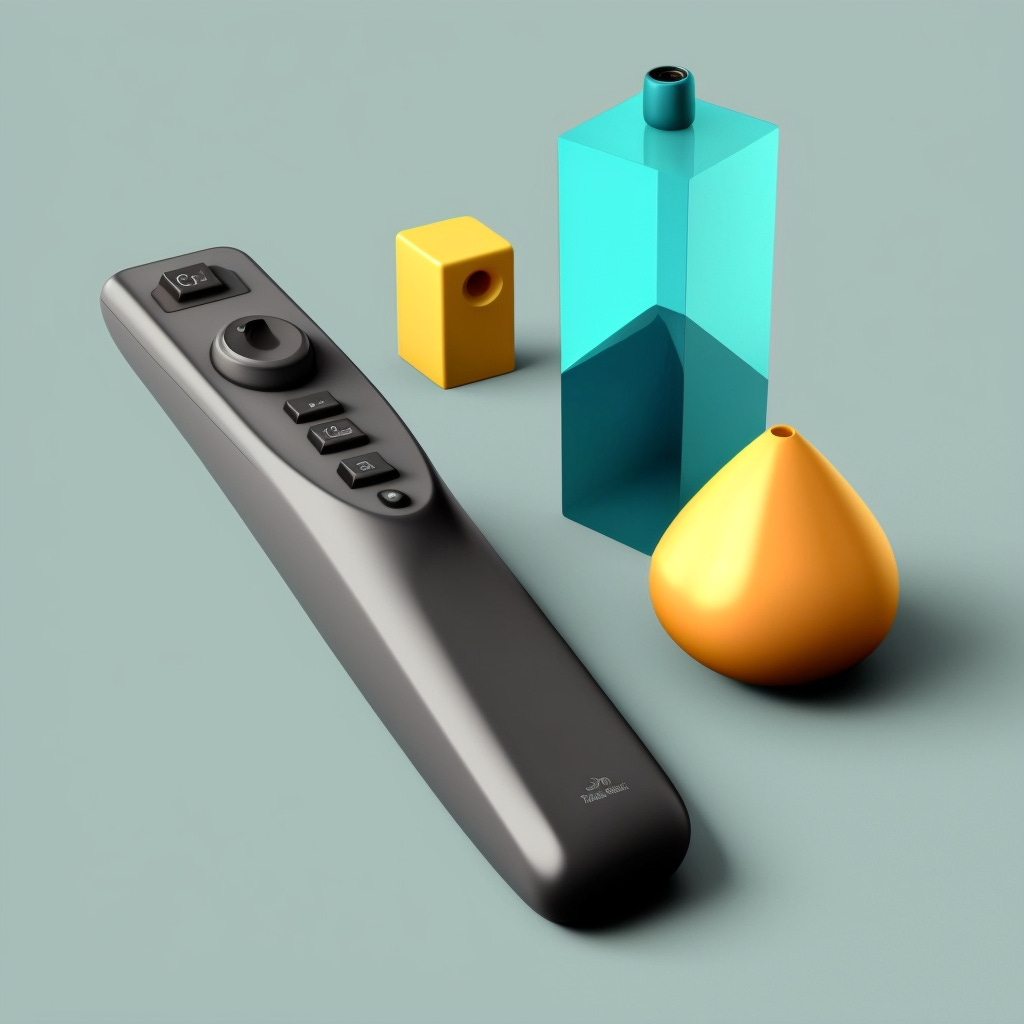The image depicts a computer-animated infographic with no text, set against a bluish-gray background. Central to the scene is a remote control, positioned diagonally toward the top left of the image. The remote has a medium gray plastic base and features four distinct buttons arranged in sequence: a small white circular button, three rectangular buttons, a larger circular dial, and another rectangular button at the top. To the right of this remote lies a yellow cube-like object with a small circle on its darker front face, possibly resembling a pencil sharpener. Adjacent to the yellow object is a larger, gradient blue block that transitions from light blue at the top to darker blue at the bottom, topped with a darker blue cylindrical lid. Completing the scene, next to the blue block, is a small golden, pear-shaped object that appears mostly orange, with its side facing the remote being a brighter yellow.